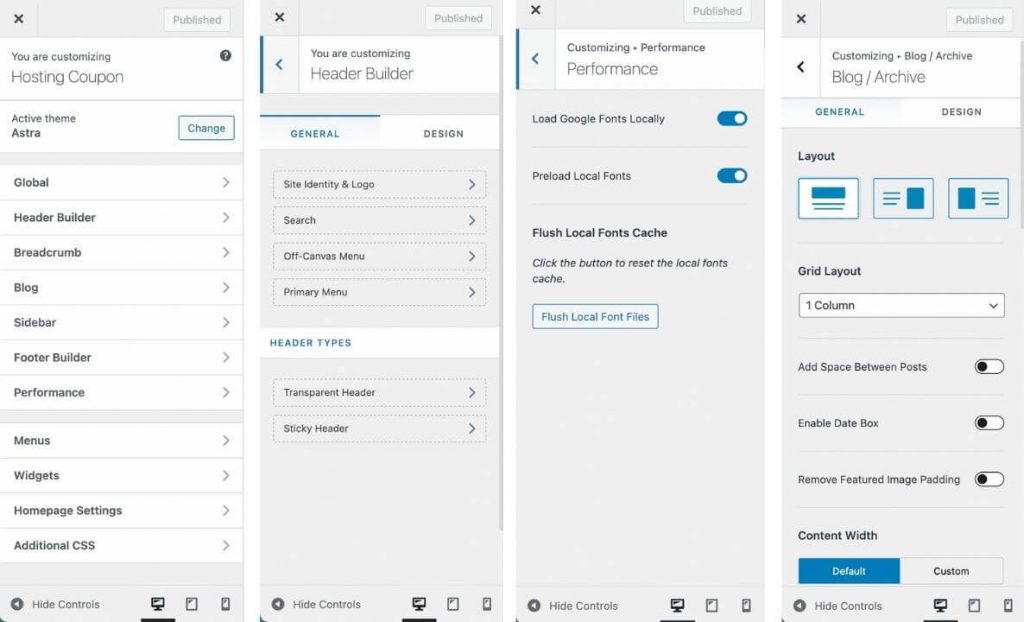This image showcases a series of screenshots detailing a step-by-step customization process, likely within a website's theme settings. The first screenshot on the left indicates that the user is interacting with a section titled "Hosting Coupon" or "Submitting Hosting Coupon," suggesting they are in the process of customizing or activating a hosting coupon feature. Below this, it mentions “Active Theme: Astra,” indicating the website is utilizing the Astra theme. Various tabs are visible, including Global, Header Builder, Breadcrumb, Blog, Sidebar, Footer Builder, and Performance, hinting at comprehensive customization options.

In the adjacent screenshot, the user has navigated to the "Header Builder" section, as indicated by the highlighted tab. Within this section, two sub-tabs, General and Design, appear, with the General tab selected. It contains various customization options such as Site Identity and Logo, Search, Off-Canvas Menu, Primary Menu, Transparent Header, and Sticky Header.

The final screenshot reveals the user has moved to the "Performance" customization settings. This section offers optimization features like "Load Google Fonts Locally" and "Preload Local Fonts," both of which are enabled. Though the exact navigation path to this page is unclear, it emphasizes the user’s focus on performance enhancements.

The sequence of screenshots provides a comprehensive look at the theme customization workflow, highlighting key sections and settings available within the Astra theme.